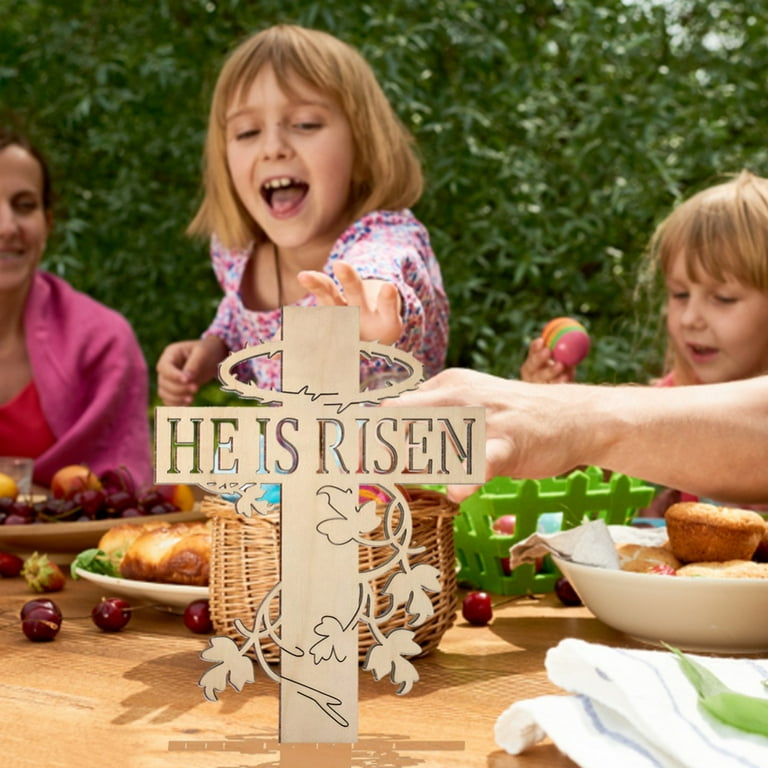This detailed photograph captures a lively Easter scene set outdoors amidst lush green foliage. The centerpiece of the image is a cross with an off-white hue, adorned with a gold inscription on its horizontal beam that reads "He is risen." This cross, which features a crown of thorns around the top, appears as an animated overlay in the middle of the photo.

Surrounding the cross is a wooden table adorned with festive food items; visible are vibrant cherries, a plate of rolls, a bowl of muffins, and a green basket likely filled with Easter treats. A wicker basket with Easter eggs also graces the table.

To the upper part of the image, a little girl with shoulder-length brown hair, dressed in a colorful, possibly tie-dye dress, reaches out towards the cross with her left hand, her mouth open as if in mid-exclamation. To her right stands another young girl, holding an Easter egg in her right hand. She has blonde, shoulder-length hair and a green plastic basket in front of her, suggesting she may be painting or collecting Easter eggs.

On the left side of the composition, partially cut off, an older woman wearing a pink jacket is seen smiling warmly, watching the children. The background is filled with a rich tapestry of trees and green leaves, enhancing the feeling of a joyful Easter celebration in an inviting outdoor setting.